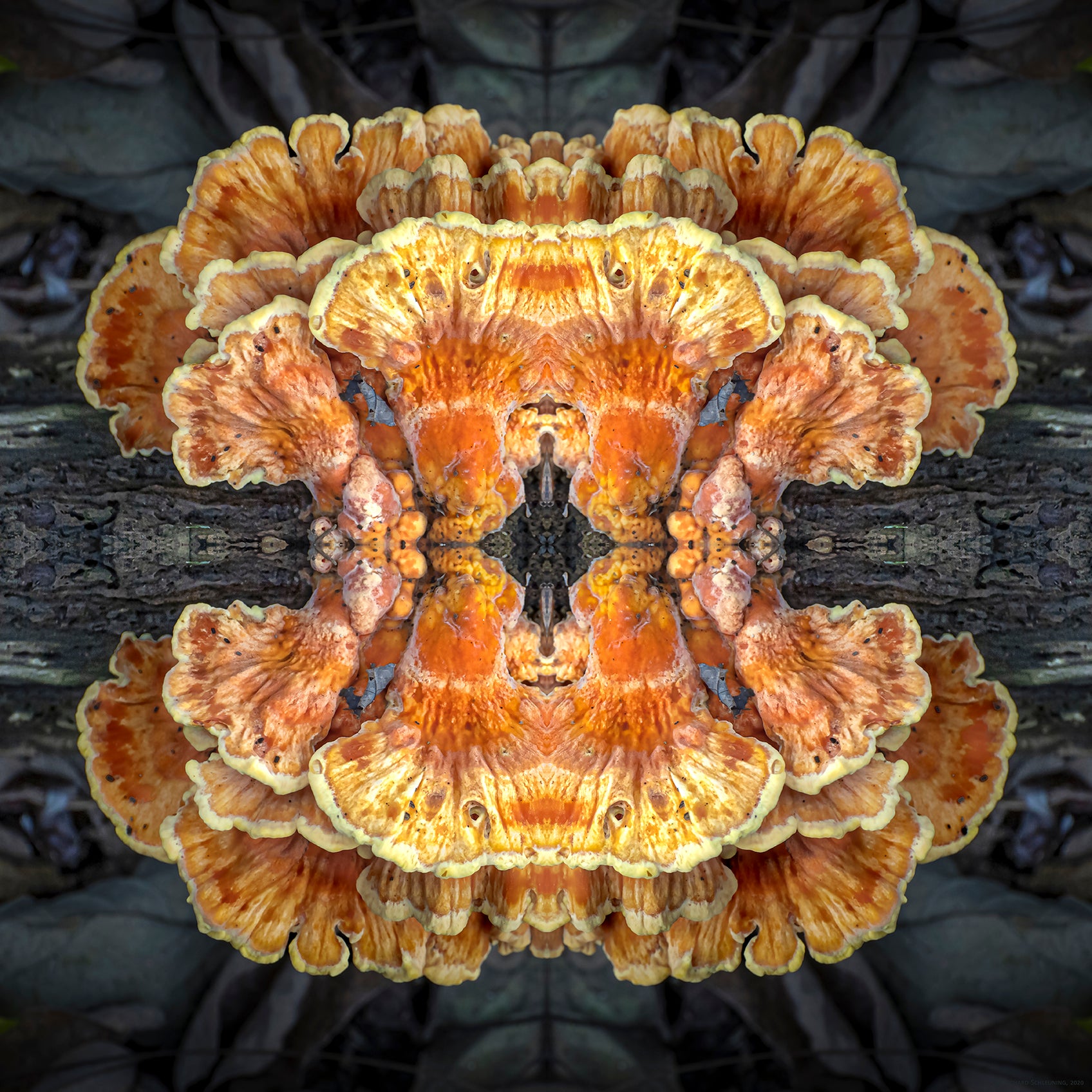The square image, set against a black background adorned with subtle gold design elements, features a vivid and intricate central design that appears computer-generated. Dominating the composition is a flared rectangular shape with rich shades of yellows, oranges, and reds, punctuated by a black center. Extending from each side of this shape are deep red accents, giving the impression of an intricate abstract design that might evoke the cross-section of coral, a sea anemone, or possibly vibrant fungi. This central motif is symmetrically reflected in a kaleidoscopic pattern, creating a mirror-like effect that radiates outwards to the edges of the image. Pops of blue and hints of pink seamlessly integrate with the overall color scheme, emphasizing the artwork's psychedelic and almost naturalistic semblance, reminiscent of a fungus or mushroom with extraordinary color variations and delicately detailed elements.